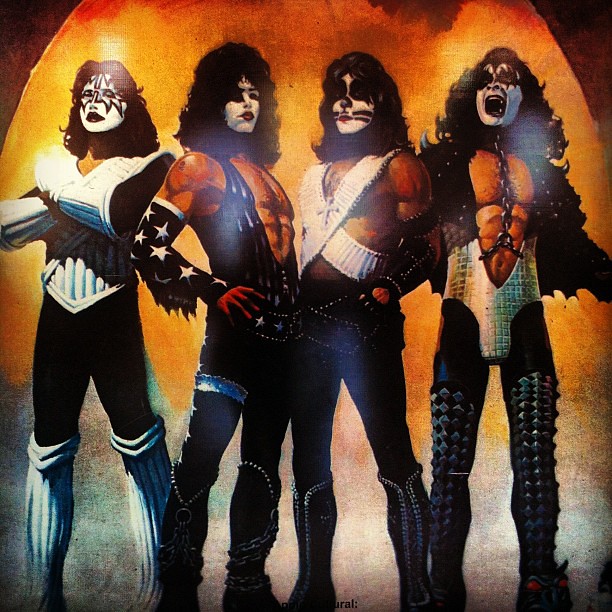The image is an artwork of the rock band Kiss, featuring four band members in their iconic concert gear, standing against a backdrop resembling an orange and red fiery sky with a misty or cloudy bottom. Each band member has long black hair and is wearing white face paint with distinctive black designs. From left to right:

- The first member wears a black outfit with white pieces crossing over his chest, white forearm cuffs, and knee-high white boots.
- The next member is clad in a black leotard with star patterns on his chest and armbands; his chest is exposed.
- The third member is dressed in an ensemble reminiscent of a cat, with black leather pants, boots, a double-crossed fabric on his chest, and face paint featuring whiskers.
- The fourth member, likely Gene Simmons, has an open chest piece, a leather jacket with spikes on the shoulders, and a large chain around his neck that attaches to his midsection. He has a fierce expression with his mouth open.

Their bizarre outfits, a mix of black leather, spikes, and some white accessories, accentuate their larger-than-life personas, reminiscent of superheroes or comic book characters. Their costumes vary from revealing chests to studded platform boots, embodying the theatrical and flamboyant style Kiss is known for.